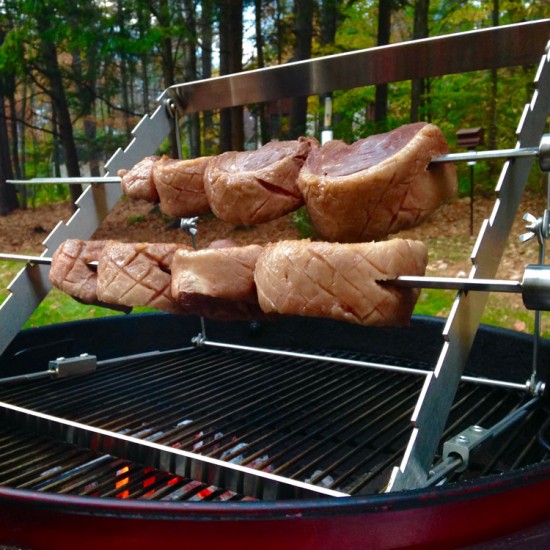This is a vibrant outdoor scene featuring a barbecue setup. The focal point is a round, red charcoal grill, with glowing coals radiating heat beneath a metal grate. Two skewers, or spits, made from long metal rods, are arranged at a slight diagonal angle over the grill. Each skewer holds around eight half-circular cuts of red meat, possibly lamb or pork, though the exact cut is uncertain. The meat on the lower skewer appears to be cooking more rapidly, possibly due to its closer proximity to the intense heat that is visibly emanating from the coals. There are subtle red flames indicating the high temperature. Behind the grill, a grassy lawn transitions into a background filled with a row of trees, their trunks thin and their leaves green and dense. To the upper right, perched on a pole just at the edge of the forest, there's a birdhouse, adding a rustic charm to the setting. The entire bottom half of the image is dominated by the grill and the skewers, emphasizing the cooking process amidst this serene natural backdrop.